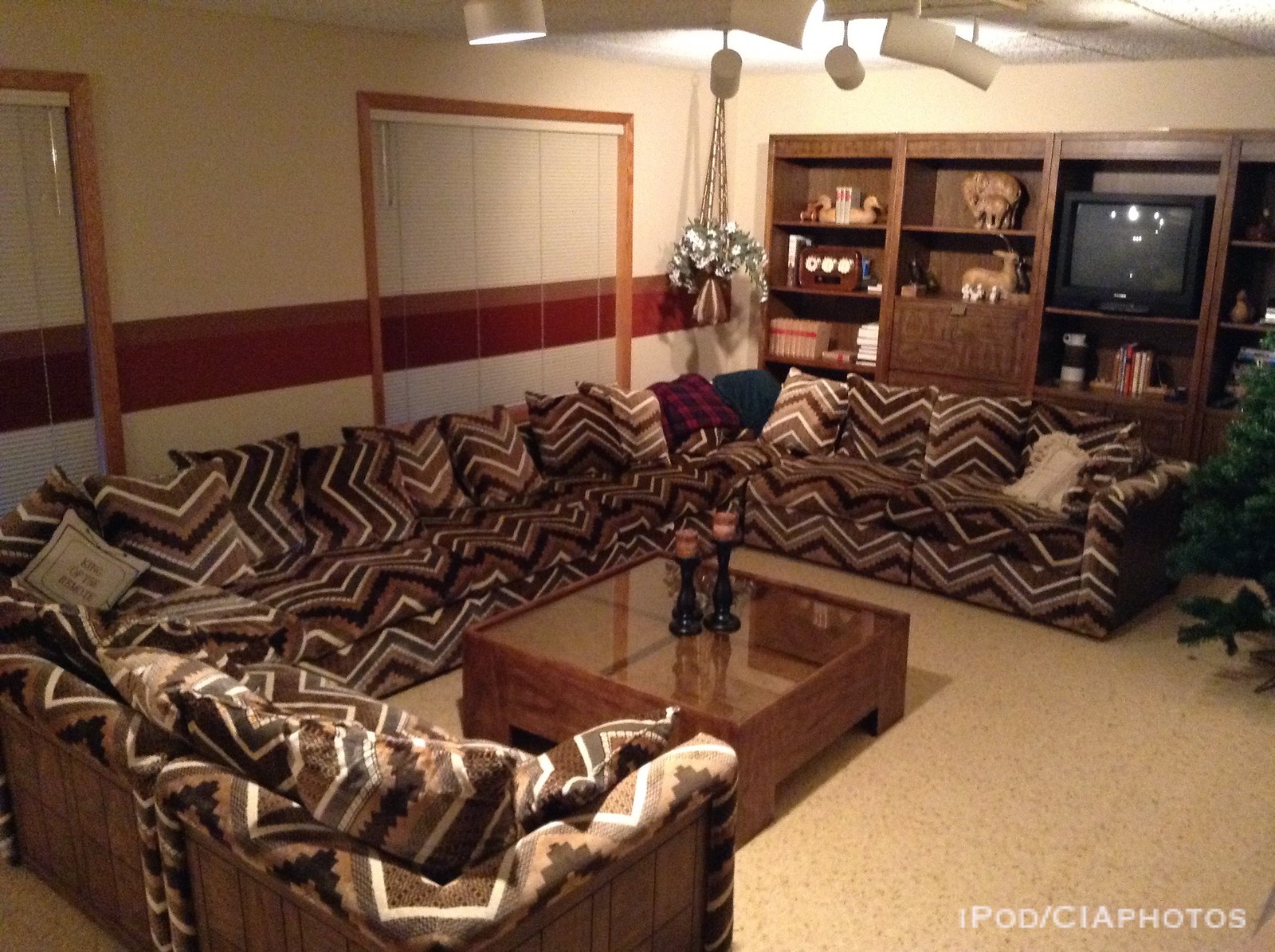This image depicts a cozy, well-decorated living room featuring a large U-shaped sectional sofa with a bold brown, white, dark brown, and beige zigzag pattern. The sectional is adorned with numerous matching pillows, except for two in the center – one with a black and red checkered pattern and the other solid dark green. A cream pillow with brown embroidered trim and some undecipherable lettering sits on the left side, and another cream pillow with fringe is on the right.

The seating area sits on a light beige carpet, centered around a square brown coffee table with a glass top. The coffee table holds two black wooden candlesticks with red and white striped candles. 

In the background on the right, there is a large entertainment unit with a retro-style bulky TV, surrounded by shelves filled with books, sculptures, and various decorative items. An adorned Christmas tree or possibly a plant peeks from the upper right corner.

The room features two windows on the left wall, each with micro blinds that seamlessly continue the room's unique horizontal stripe pattern of dark red and light brown, which also extends across the walls. The walls are painted a creamy off-white with these distinctive horizontal stripes.

Enhancing the room's subtle sophistication, white track lighting is mounted on the ceiling which is complemented by ceiling tiles. Additionally, a hanging planter with beautiful white flowers adds a touch of nature and freshness to the space. The floor is covered with light cream carpet that may also be linoleum, completing the room's warm and inviting ambiance.